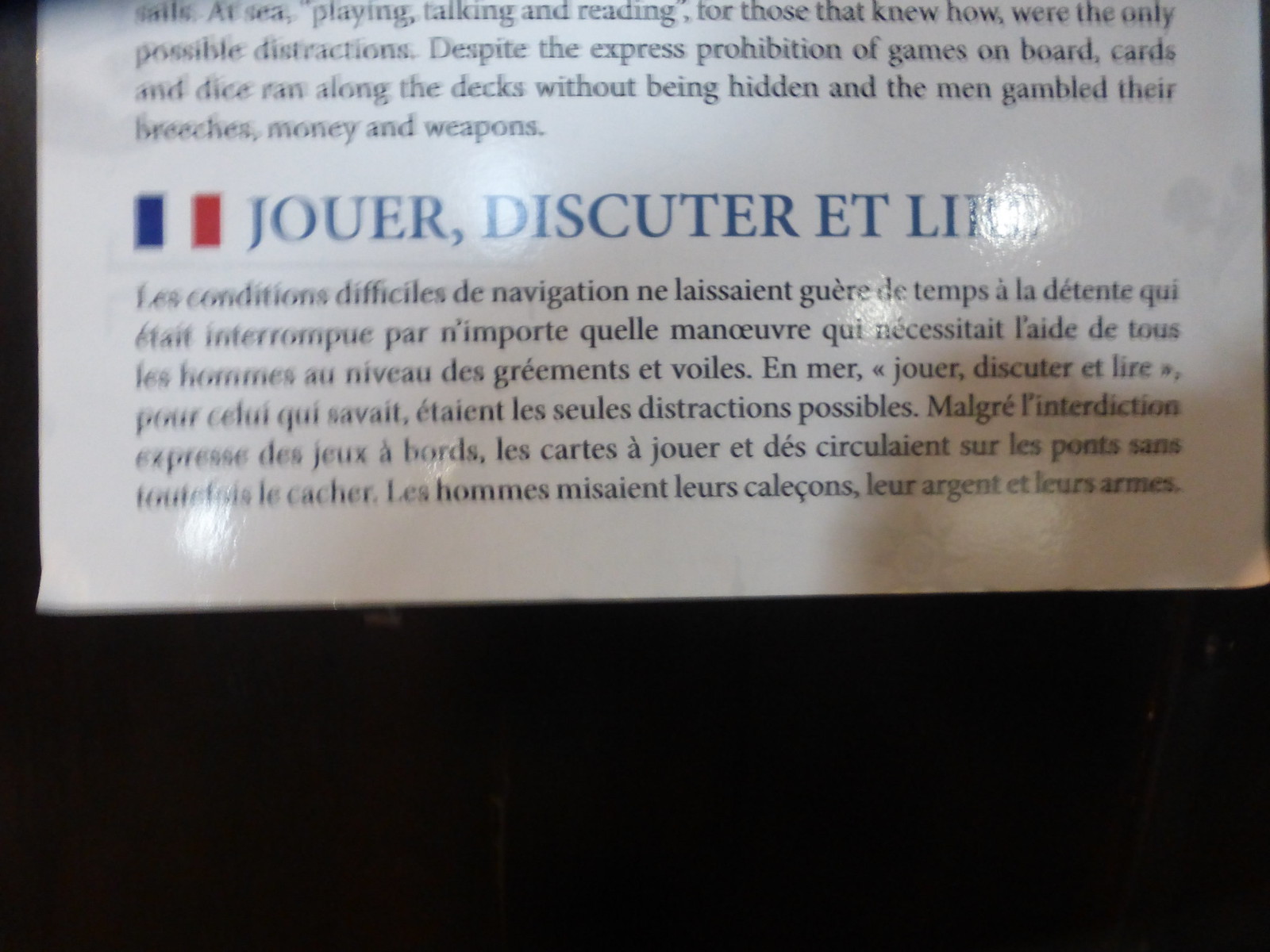This is an intricately detailed, color photograph of an informational poster or plaque, presented in landscape orientation. The plaque, positioned within the upper half of the image, is set against a predominantly black background which occupies the lower portion of the frame, giving the impression of a dark room or indoor setting. The photograph appears slightly wider and a bit taller than a high-definition TV screen.

The poster itself displays two paragraphs of text in two different languages. The first paragraph, written in English, is situated at the upper section and is partially cut off at the top. It describes a scenario, with the last visible sentence reading: "Despite the express prohibition of games on board, cards and dice ran along the decks without being hidden and the men gambled their breaches, money, and weapons." 

Below the English text, there is a title in French, displayed in underlined bold blue letters adjacent to the French flag, showcasing its iconic red, white, and blue horizontal stripes. Beneath this, a paragraph in French follows, written in black text. The entire object, possibly a memorial plaque on a ship, is set against a stark black background with no additional objects or embellishments, emphasizing the text's importance and solemnity. The visual details indicate a photographic realism style, capturing the essence and context of the plaque with precision.